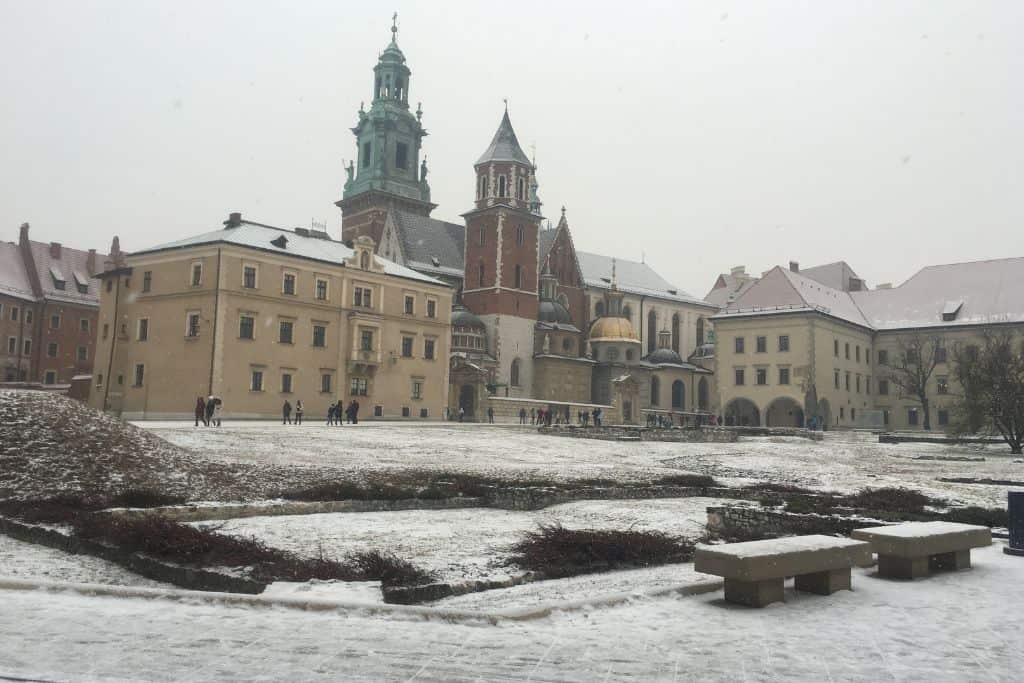This photo showcases a snowy urban landscape dominated by a collection of various buildings exhibiting diverse architectural styles and colors. At the center, a tall, ornate tower with a mini-dome and spear at the top stands out, flanked by two three-storied brown buildings. The tower features two rectangular windows in its upper echelons. Surrounding the tall tower are buildings characterized by decorative architecture; some have widow's peaks and ornamental weathervanes. The buildings range in color from beige and tan to red and brick, with roofs of differing hues. One prominent building has long vertical windows and another is made of clay-colored stone. There are brown benches, likely made of concrete, scattered throughout the snow-covered foreground. People are seen walking along the stone paths near the buildings, adding life to the otherwise still, wintry scene. In the distance, some trees and red vegetation break up the urban expanse, which is devoid of any labeling text.